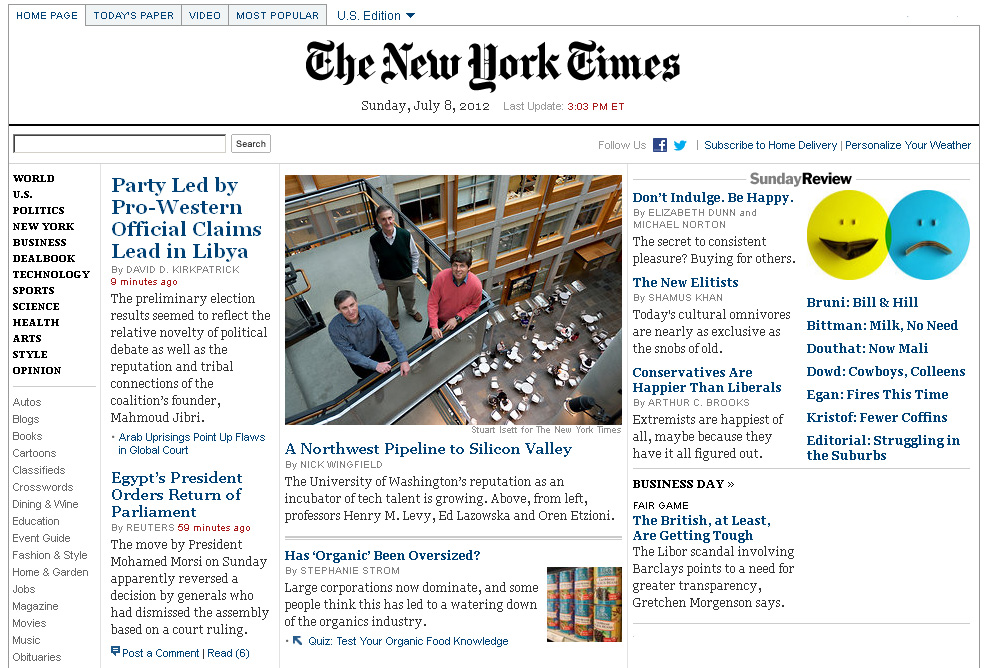This is the front page of The New York Times, dated Sunday, July 8, 2012, with the last update at 3:03 PM ET, and it is labeled as the U.S. edition. The iconic "The New York Times" title is prominently displayed in script across the center. Below this header, the date and time of the last update are clearly printed.

On the left-hand column, highlighted categories include: World, U.S., Politics, New York, Business, DealBook, Technology, Sports, Science, Health, Arts, Style, and Opinions. There are also non-highlighted options such as Autos, Classifieds, Education, and Movies.

To the right, various headlines capture the reader’s attention. First, "Party led by pro-Western official claims lead in Libya" and "Egypt's president orders return of parliament" are the prominent news stories. 

Occupying a central position on the page is a photograph taken indoors featuring three men. The scene depicts them standing on a balcony, looking upward at the camera with smiles on their faces. In the background stands a middle-aged man wearing a vest. In the foreground, a younger man in a long-sleeved blue shirt and another man in a red shirt are visible. Below the balcony, tables and chairs are scattered around, with people seated at some of them.

Additional headlines include: "A Northwest pipeline to Silicon Valley," "Has organic been oversized?" and a series of intriguing articles such as "Don’t indulge, be happy," "The new elitist," "Conservatives are happier than liberals," and "The British, at least, are getting tough."